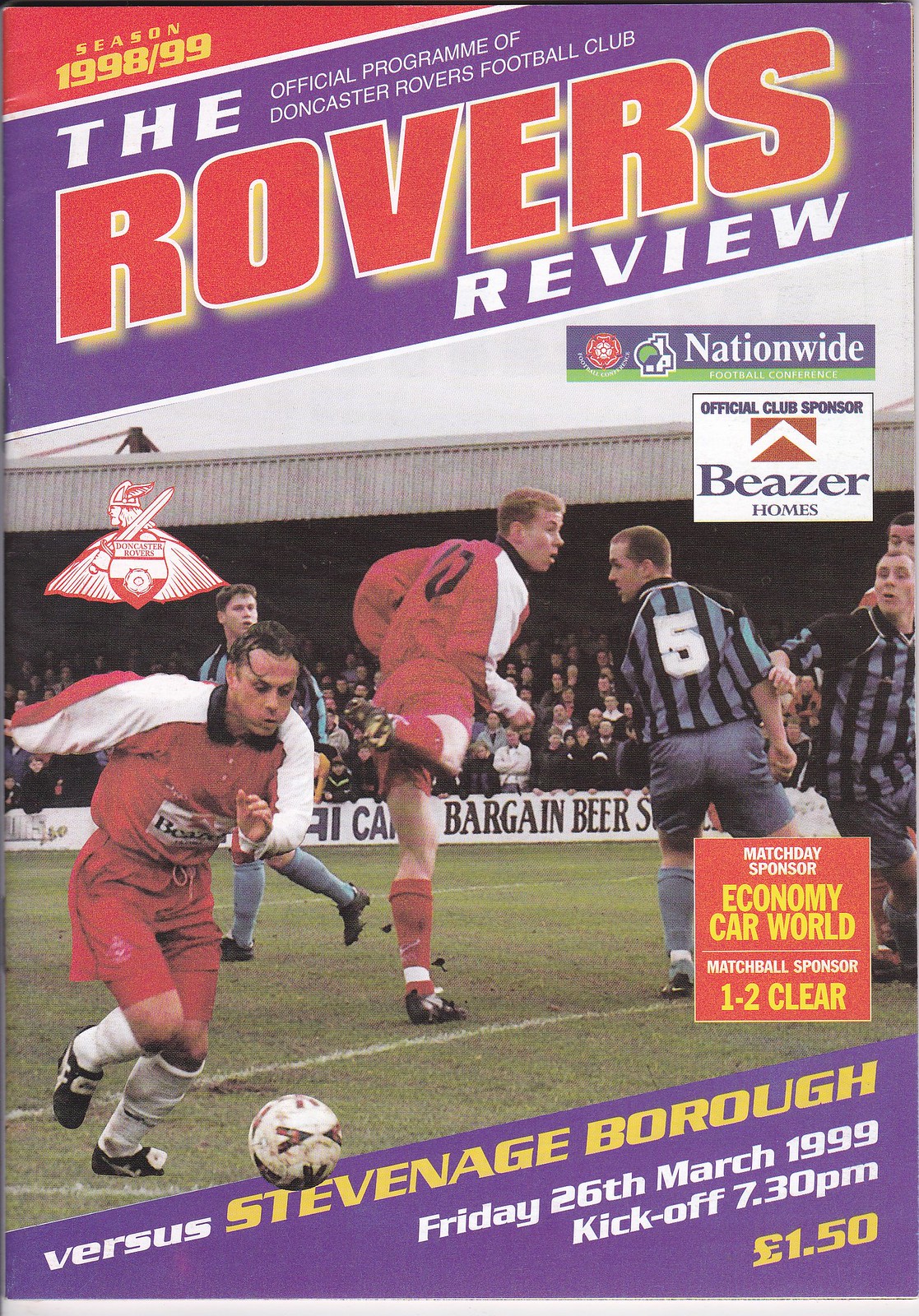The cover of the 1998/99 Doncaster Rovers Football Club official program features a blend of vibrant graphics and dynamic action photography. At the very top left corner, a red rectangle with yellow text prominently announces "Season 1998/99." Below this, a purple banner stretches across the top, displaying "The Official Program of Doncaster Rovers Football Club" in small white text. Centrally placed within this banner, "ROVERS" stands out in bold, red text with white and yellow borders, followed by "Review" in white text.

Dominating the middle of the cover is a vivid action photograph. The image captures an intense soccer match on a green field, slightly worn with patches of dirt and clear white lines. Two teams are in play: one in red jerseys with white shoulder stripes and red shorts, and the other in dark blue and black vertical stripes with gray shorts. A notable player in dark uniform, bearing a white '5' on the back, is positioned near the center right of the image, while a player in red hustles towards the soccer ball in the foreground. The background reveals spectators seated in the stands beneath a silver stadium roof against an overcast sky. 

Scattered around the cover image are various sponsor logos. The bottom of the photograph features a red logo that reads "Match Day Sponsor, Economy Car World" alongside "Match Ball Sponsor, 1-2 Clear." The top of the image has a black square stating "Official Club Sponsor Beezer Homes," with another logo above this that reads "Nationwide" in white text on a purple background.

In the bottom right corner, a triangular purple banner provides specific match details in a mix of white and yellow text: "Versus Stevenage Borough, Friday 26 March 1999, kickoff 7.30 p.m." with "150 pounds" highlighted in yellow. The overall composition of the magazine cover is a detailed and engaging preview of the match day experience, capturing the essence of Doncaster Rovers Football Club's 1998/99 season.